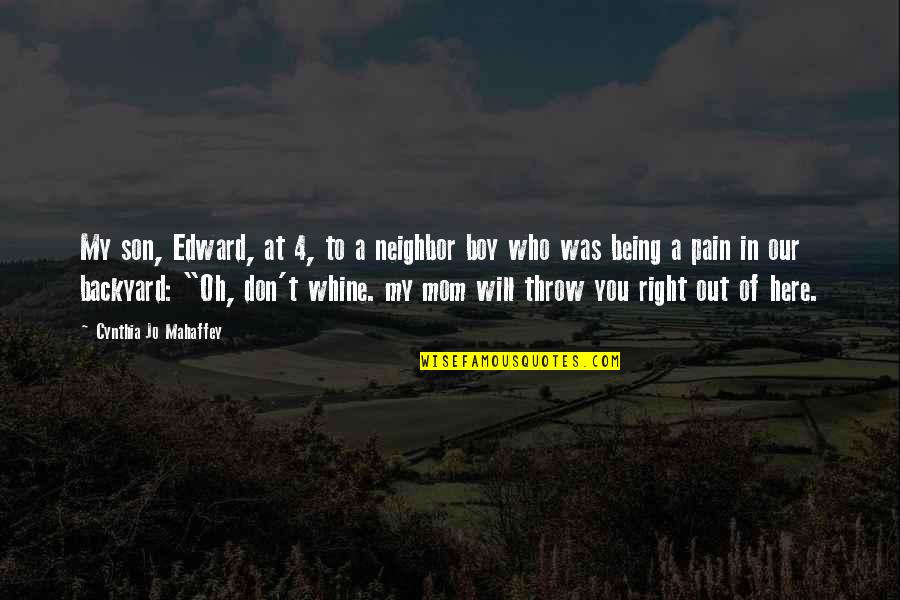An image featuring a dimly lit, natural landscape from an elevated viewpoint, revealing a verdant field with scattered plants, trees, and a winding road. Above the expanse, a cloud-laden sky with patches of light blue peeks through. The photograph, enveloped in a darker tone, serves as the backdrop for a prominently displayed quote in bright white text centralized in the middle of the image: "My son Edward, at four, to a neighbor boy who was being a pain in our backyard, 'Oh, don't whine. My mom will throw you right out of here.'" The quote is attributed to Cynthia Jo Mahaffey, with her name positioned just below the text, and further down, a small yellow rectangle contains the source, wisefamousquotes.com.